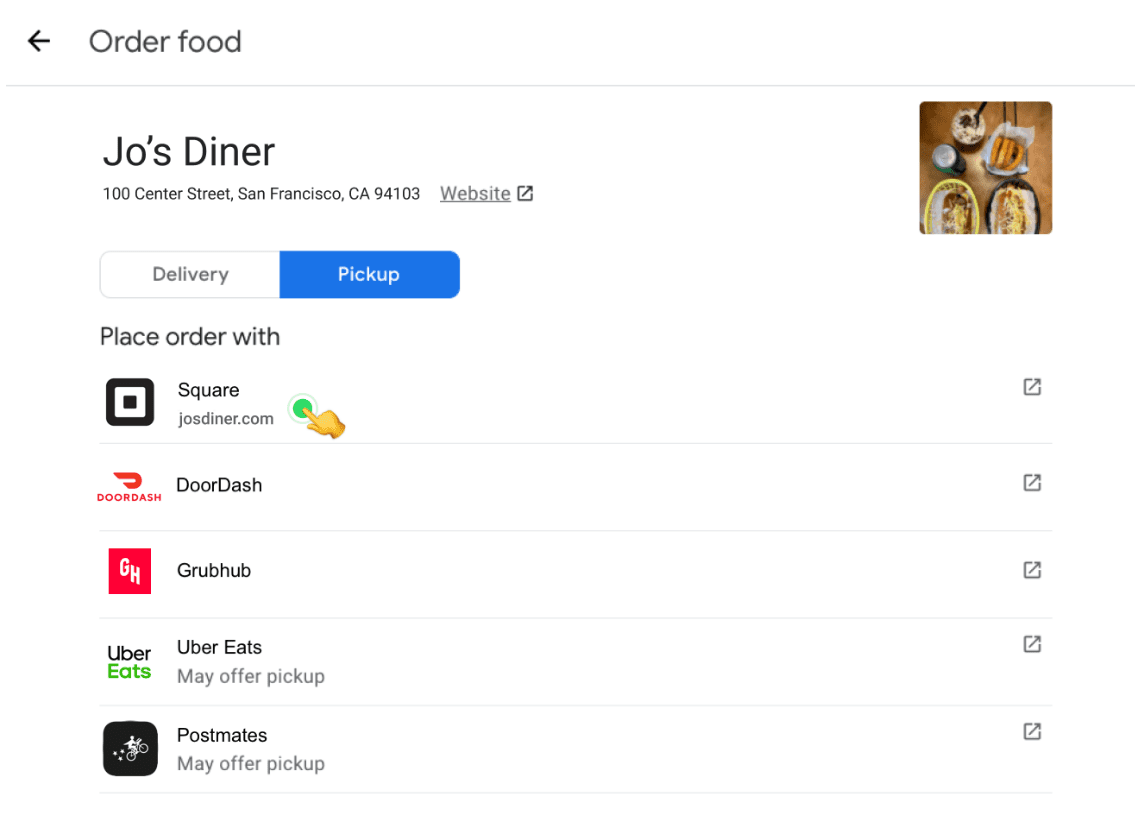The image features a user interface from an online food ordering platform with a white background. In the top left corner, there is a black left-pointing arrow followed by the text "Order Food" in black. Below this, a grey divider line separates the header from the main content.

Prominently displayed in bold black letters, "Joe's Diner" appears, with the address "100 Center Street, San Francisco, CA 94103" written in smaller black text underneath. Next to this, an underlined "Website" link is accompanied by an icon of a box with an arrow pointing to the top right corner, indicating an external link.

To the right, there is an image set against a brown background showcasing several wraps or sandwiches. The wraps are white, presumably paper-wrapped, and reveal colorful fillings featuring shades of pink, brown, and yellow.

Below and to the left, there are two buttons: one for "Delivery" in black text with a rounded design, and another for "Pickup" in white text on a blue background. Further down, the text "Place order with:" is followed by a list of available delivery services: Square, DoorDash, Grubhub, Uber Eats, and Postmates, each with their respective logos. The text "may offer pickup" appears in grey under the Uber Eats and Postmates options.